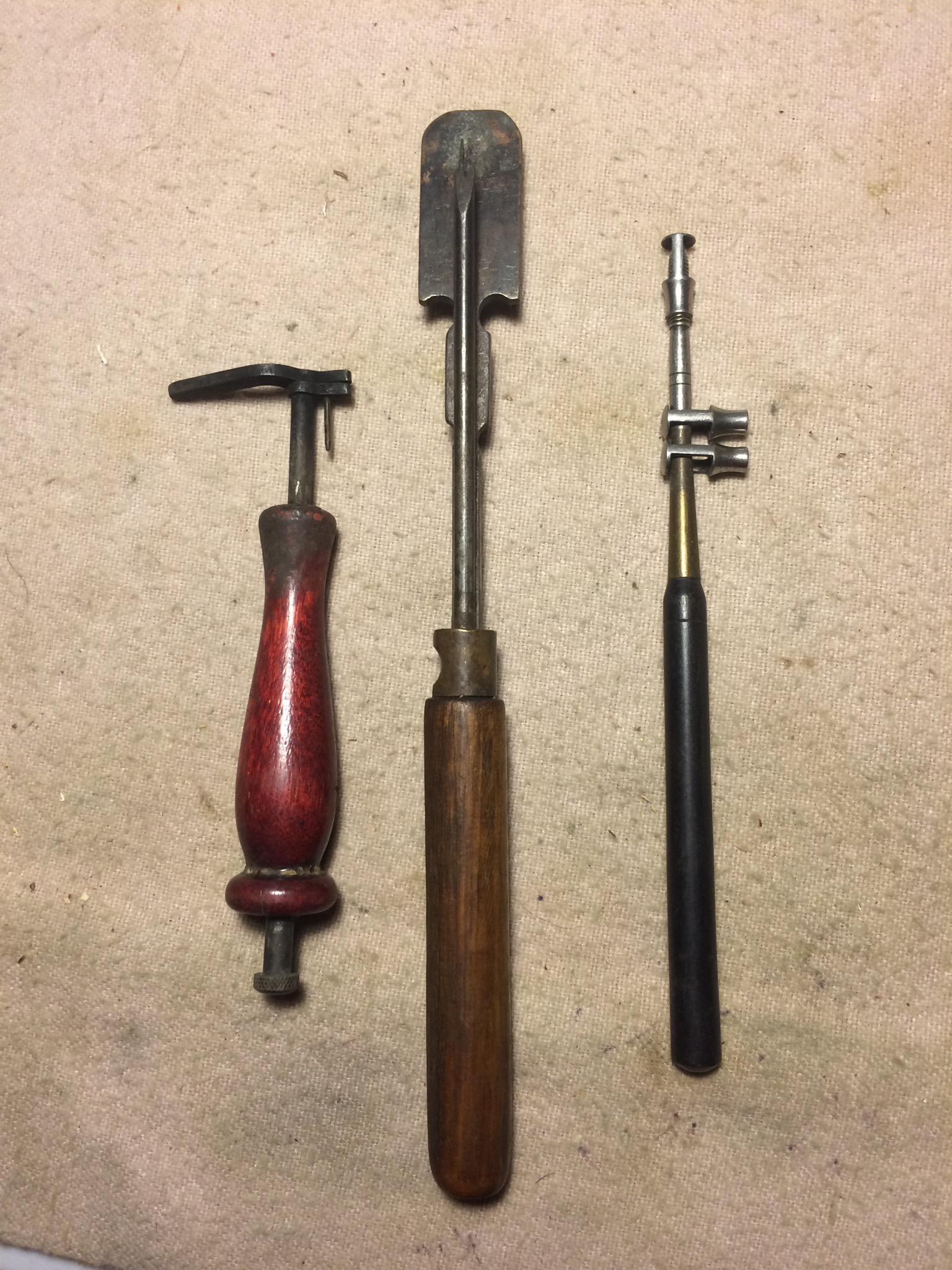This detailed photograph showcases three distinctive vintage tools meticulously laid out on a slightly dirty, tan cloth. 

On the left, there's a compact tool featuring a thick, subtly contoured handle crafted from rich, red or maroon wood. A sturdy vertical metal rod pierces through the handle, capped with a unique dark metal piece resembling a flattened spout or hoe, while a round metal element anchors the bottom.

Dominating the center, the longest of the trio, is a tool with an elongated brown wooden handle. This handle tapers into a slender metal shaft that expands into a shovel-like, paddle-shaped tip, suggesting a specialized digging or scraping function.

The tool on the right is the thinnest and sports a sleek black handle. Extending from this handle is a metal shaft with a gold-to-silver gradient, culminating in a flat, screw-like tip. Intriguingly, two additional silver metal pieces with similar screw-like ends protrude horizontally at a 90-degree angle from the main shaft, adding to its peculiar design and potential utility.

Each tool's metal components are oriented upwards, juxtaposed against the earthy-toned fabric, which serves as a muted backdrop highlighting their distinctive features and aged craftsmanship.